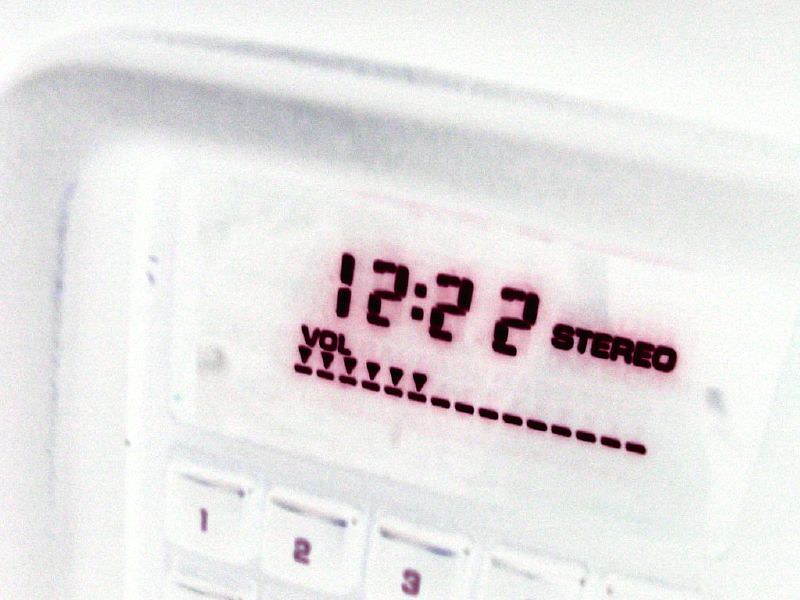On a grainy and fuzzy white background, a rectangular device is centrally displayed, bordered evenly on all sides. The digital screen on the device prominently shows "12:22" in black numbers, followed by "STEREO" in bold black font. Below the display on the left side, the word "Volume" is inscribed with an array of six downward-pointing arrows beneath it, leading to a dotted line that spans horizontally. Towards the bottom, there are large white buttons labeled with numbers "1," "2," and "3," with another indistinct button possibly marked in red. The overall image appears to have a filter applied, making everything but the digital display appear washed-out, thus causing the screen to stand out strikingly against the white backdrop.